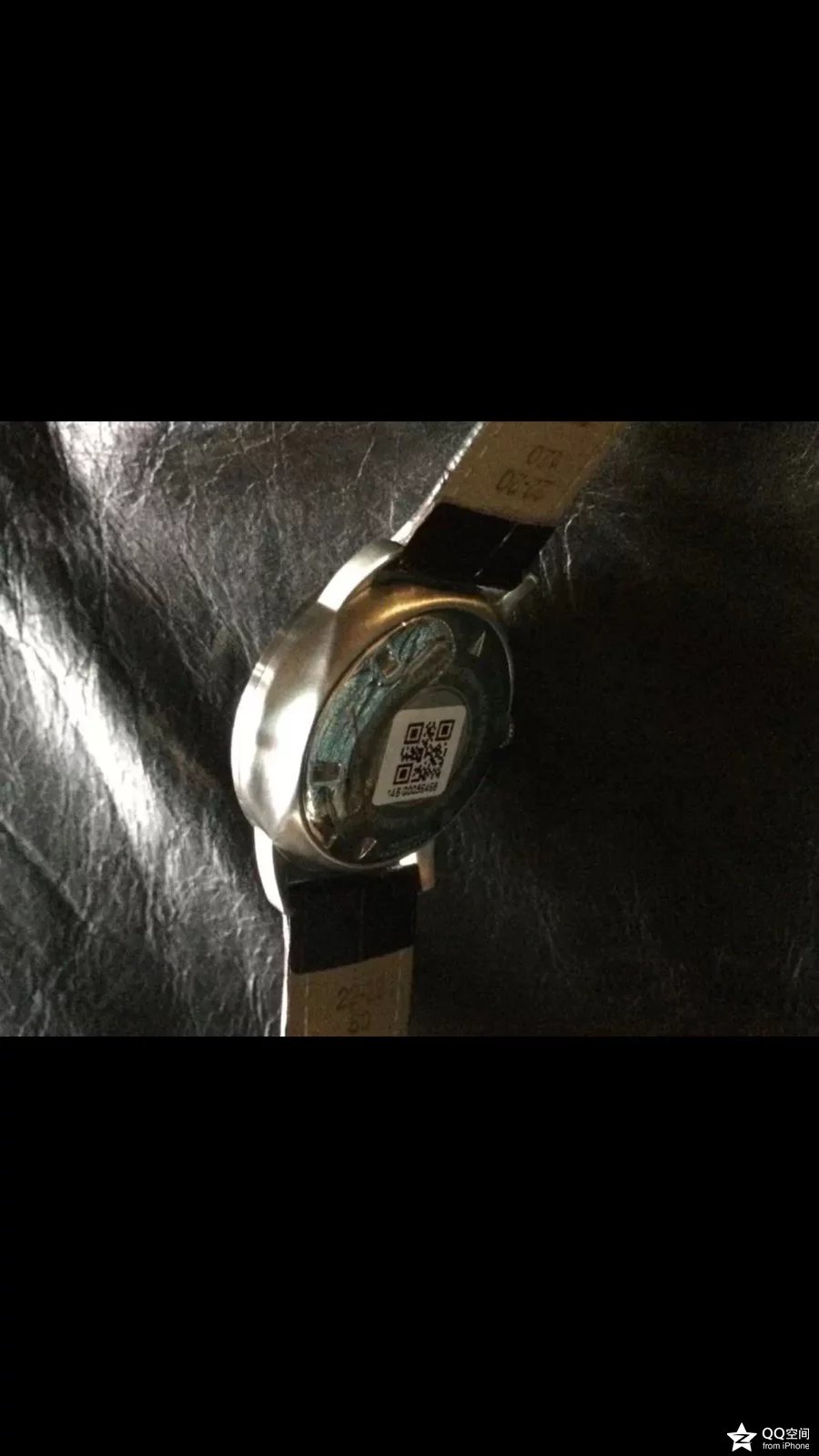The image depicts a dimly lit, close-up photograph of a watch resting on a textured, worn black leather surface with white crumples. The focus is on the back of the watch, which is metallic silver in color. The watch face is angled towards the top-left corner of the frame. The lower portion of the watch features a glass section that reveals some interior components, and a white label with black writing is placed on the glass, possibly featuring a QR code.

The watch bands are prominently shown: the upper band extends towards the top-right, while the lower band stretches downwards. Both bands have black markings followed by brown segments, and the numbers "2250" and "2220 50" can be seen on the lower and upper bands respectively, though some of the text appears blurry.

In the bottom-right corner of the photograph, there is a small lock icon and a white star with the letter 'T' inside it, accompanied by tiny text saying "DQSM". The overall dimness of the lighting and muted colors add to the detailed, intricate appearance of the watch and its setting.